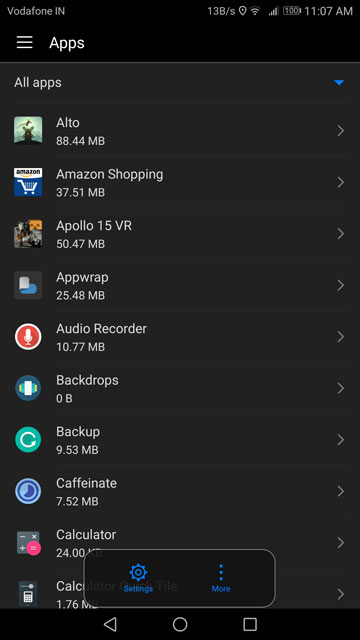This is a detailed description of a mobile phone screenshot:

The screenshot displays a mobile phone interface in dark mode, featuring a charcoal gray background. At the top of the screen, a black bar with white font provides important information. On the left corner of this bar, it indicates the network carrier, "Vodafone," while the right corner displays the current time, "11:07 a.m." The status icons show a fully charged battery, 100% Wi-Fi signal, and full mobile signal strength, along with a relatively slow data speed of "13 B/s."

Below the black bar, the interface displays the word "Apps" in white font, accompanied by three small horizontal bars stacked on each other to the left, also in white. Scrolling down, the text "All Apps" in white font appears on the charcoal gray background, with a small blue downward arrow to its right, indicating the presence of a dropdown menu.

The main content of the screenshot comprises a list of the user's apps, each labeled with its respective data size:

1. **Alto** - 88.44 MB
2. **Amazon Shopping** - 37.51 MB
3. **Apollo 15 VR** - 50.47 MB
4. **App Wrap** - 25.48 MB
5. **Audio Recorder** - 10.77 MB